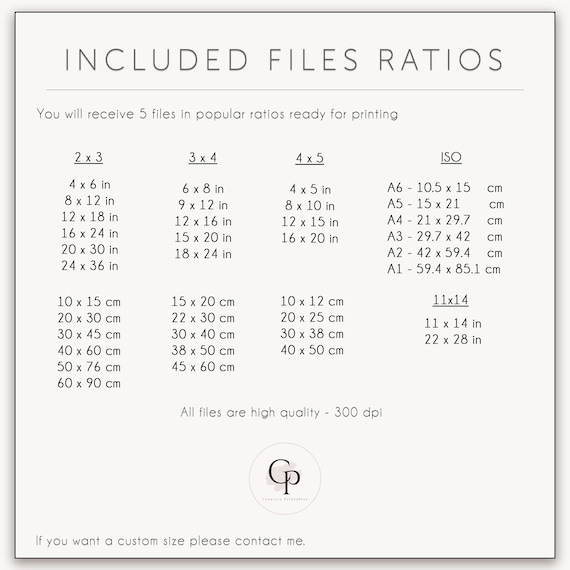This image is an advertisement for included file ratios, designed as a detailed worksheet. The top section features a white background with black edges and begins with a title that reads "Included File Ratios." A thin black line separates this heading from the main content below. The ad states, "You will receive five files in popular ratios ready for printing," followed by four different columns listing sizes in both inches and centimeters: 2x3, 3x4, 4x5, ISO, and an additional 11x14. Each ratio includes different multiples, such as 2x3 extending to 4x6 and 8x12, and 3x4 to 6x8 and 9x12. Underneath the columns, it notes that "All files are high quality - 300 DPI." At the bottom left, there's a call to action: "If you want a custom size, please contact me." The company's logo—a crest with the letters "CP" in a circle—appears just above this text.